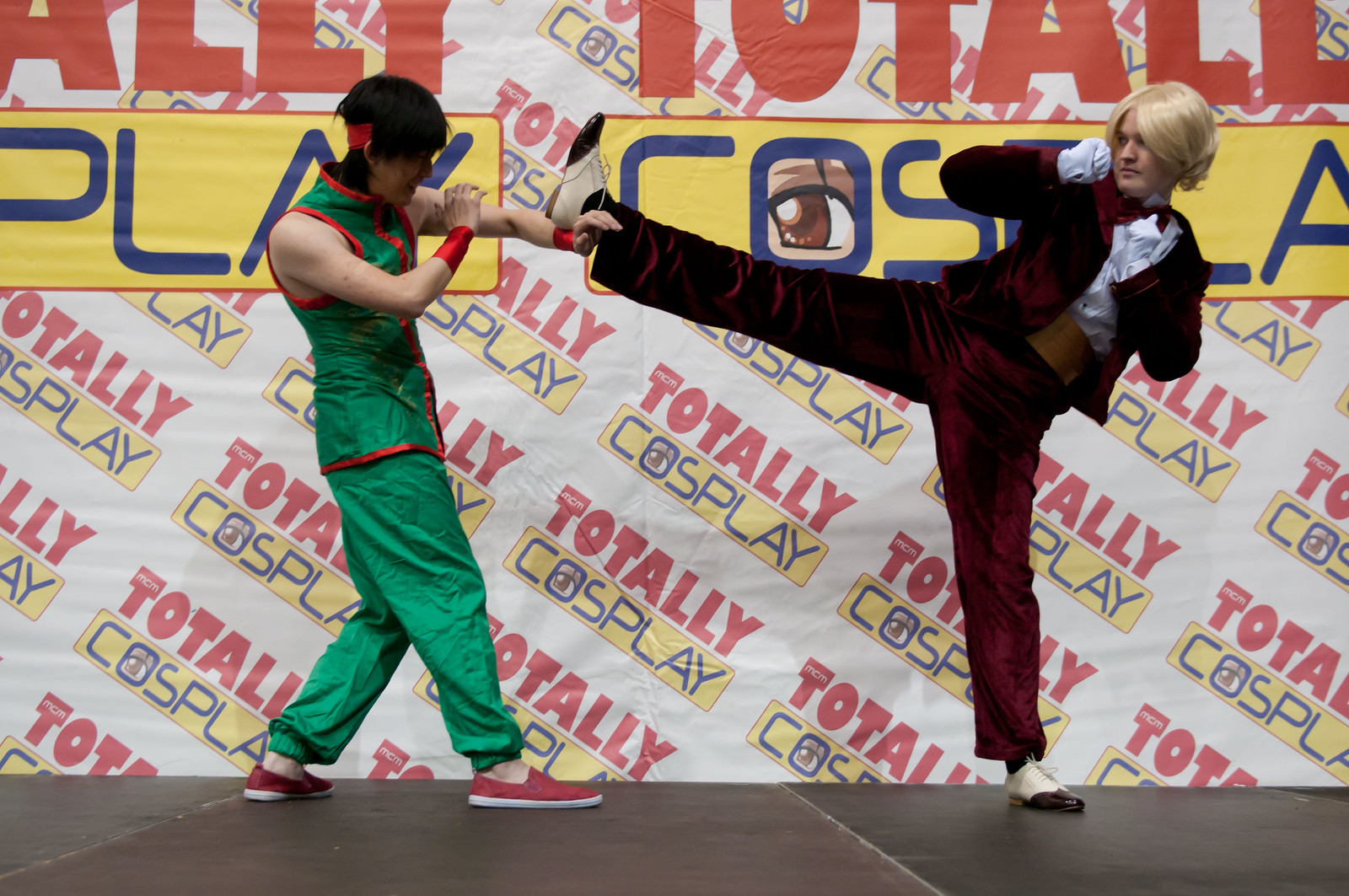In this detailed photograph, taken indoors and rectangular in shape, we see a dynamic scene set on a flat, gray stage. The backdrop is dominated by a large banner that repeatedly features the words "Totally Cosplay" in bold red and blue letters on a yellow background, arranged both horizontally at the top and in diagonal rows from the lower left to the upper right. 

On the left side of the stage stands a man with straight black hair, tied back with a red headband. He is clad in a sleeveless green and red Chinese-style costume, featuring red trims and red shoes. He stands in a defensive posture, his arms raised to block an incoming attack. 

On the right side, another individual with a yellow wig and light skin wears a dark red, silky velvet costume, complemented by a white undershirt, white gloves, and black and white spats. He is captured mid-action, performing a high martial arts kick aimed at the man on the left. The scene is evocative of a dynamic moment from a fighting game, set against the visually busy yet thematic "Totally Cosplay" backdrop, emphasizing the event’s vibrant cosplay culture.